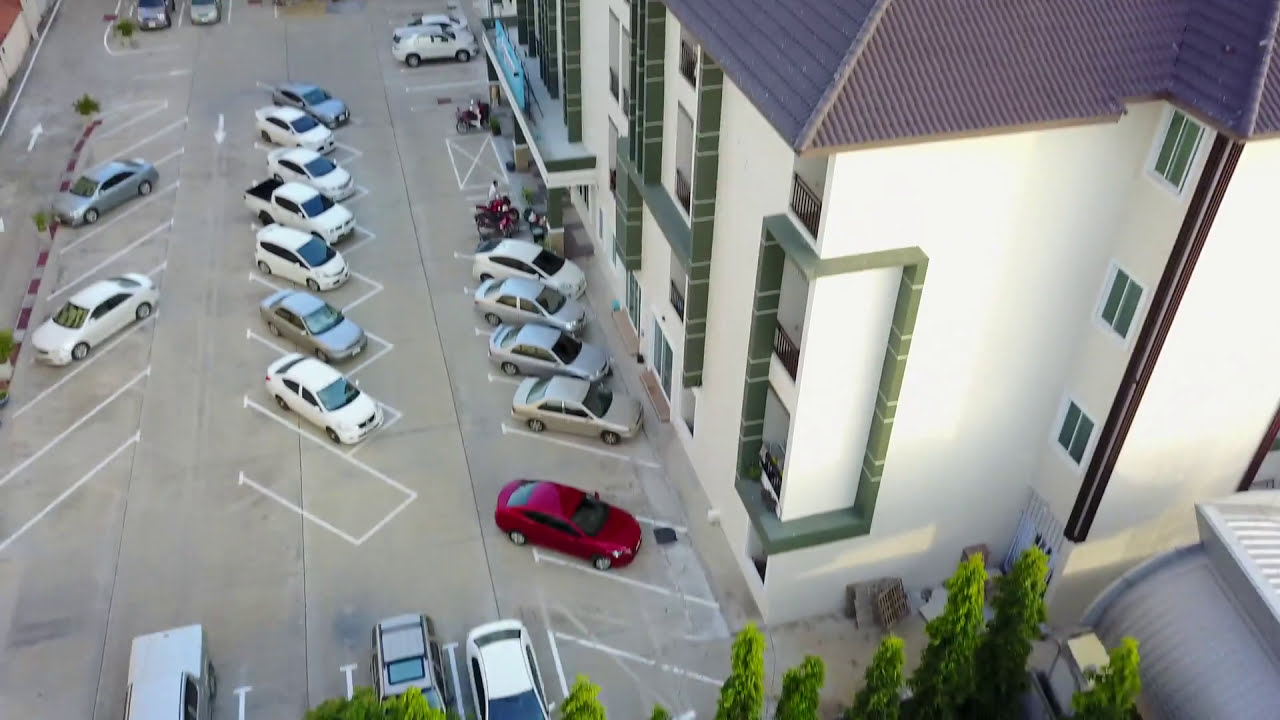In this aerial photograph, taken from a high vantage point such as a drone, an upper window, or a roof, the perspective reveals a detailed view of a tall, white building adorned with green framing in seemingly random blocks. This structure, which could be an apartment complex, hotel, or motel, features several balconies and uniformly arranged rows of windows. The building is surrounded by a sizable parking lot that occupies roughly half of the image. Within this parking area, most vehicles are white or gray, with the notable exception of a single bright red car and a couple of motorcycles. The parking spaces are laid out diagonally, and although the lot is substantially filled, there are still a number of available spots. The paved surface of the parking lot is a grayish-brown, with clearly marked white arrows and parking spot outlines. In the foreground, only the tops of a few trees are visible, suggesting they are quite tall.